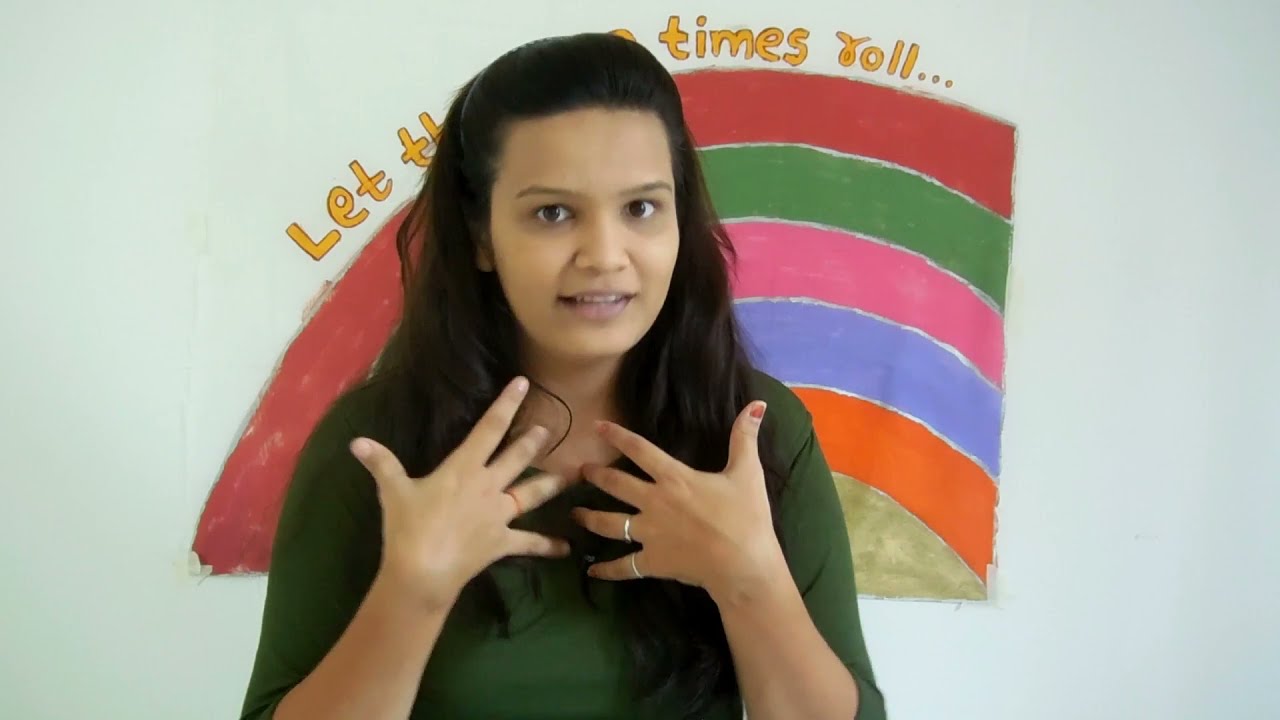The image features a young girl with brown skin and long, dark brown hair that drapes to her chest, pulled back from her face with a headband or hair clip. She wears a green, elbow-length sleeved top and stands in front of a faded white wall adorned with a rainbow painting. The rainbow artwork includes vibrant colors: red, green, pink, purple, blue, orange, and yellow, and appears to have been created by a young or emerging artist. Visible behind her are the orange words with a black outline, "let... t... times roll," suggesting the full phrase "let the good times roll." Her expressive brown eyes gaze forward, and her mouth is slightly open, showing the top row of her teeth. She holds her hands up in front of her chest, fingers spread out. The right hand has a silver ring on the ring and pinky fingers, with the thumb painted red. The left hand features another ring on the ring finger, also painted red. The backdrop below the rainbow painting is blotchy brown, enhancing the intricate details of the scene.